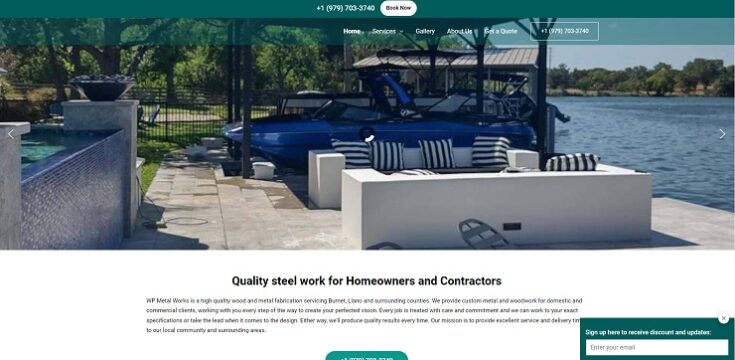The website page features a serene and inviting lakeside scene, although the company name is not indicated. At the top of the page, there's a phone number and a prominent "Book Now" button. Below these, navigation options are listed: Home, Services, Gallery, About Us, Get a Quote, and the phone number is repeated.

The main image showcases a tranquil lake with a solid cement dock adorned with stylish outdoor furniture. The furniture set includes white seating with blue and white striped pillows, creating an inviting relaxation area. Nearby, two boats are moored—the first is a blue boat with a canopy top, and the second, partially obscured, appears to be black and white. To the left, the edge of a swimming pool is visible, framed by a wrought iron fence and lush trees, suggesting a luxurious and comfortable outdoor environment.

On the right side of the image, a portion of the lake is visible, leading to a distant shore lined with trees. Below the picture, a bold caption reads, "Quality steel work for homeowners and contractors." The section underneath contains additional informational text, while a sidebar on the right offers visitors the opportunity to sign up for contact updates or discounts.